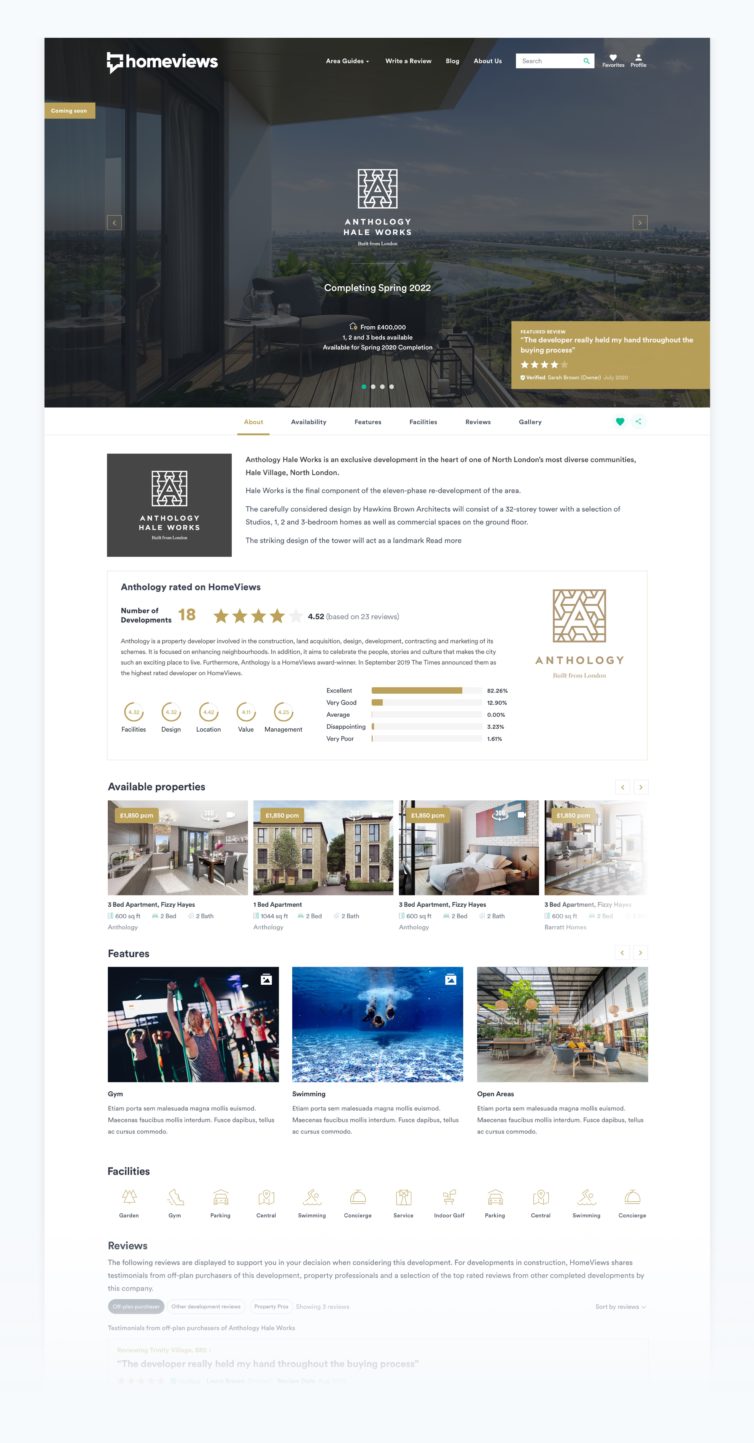The website page of Anthology Haleworks is challenging to read, even when enlarged. The page appears to represent a real estate company, offering a variety of properties. The top of the page is dominated by a blue and gray box featuring the text: "Home Views, Anthology Haleworks, Completing Spring 2022." Scrolling down, there is a section titled "Available Properties," accompanied by seven images. 

The first image depicts a meeting room furnished with sleek, gray furniture. The second image showcases two beige buildings, possibly residential or commercial properties. The third picture presents a luxurious hotel-like room with a double or king-size bed. The fourth image is indiscernible. In the fifth picture, people are seen working out in a gym, highlighting the fitness amenities available. The sixth image portrays an underwater scene with vibrant blue colors, featuring fish, suggesting an aquarium or water-related facility. The final image displays a spacious open area with tables and plants, ideal for social gatherings or meetings.